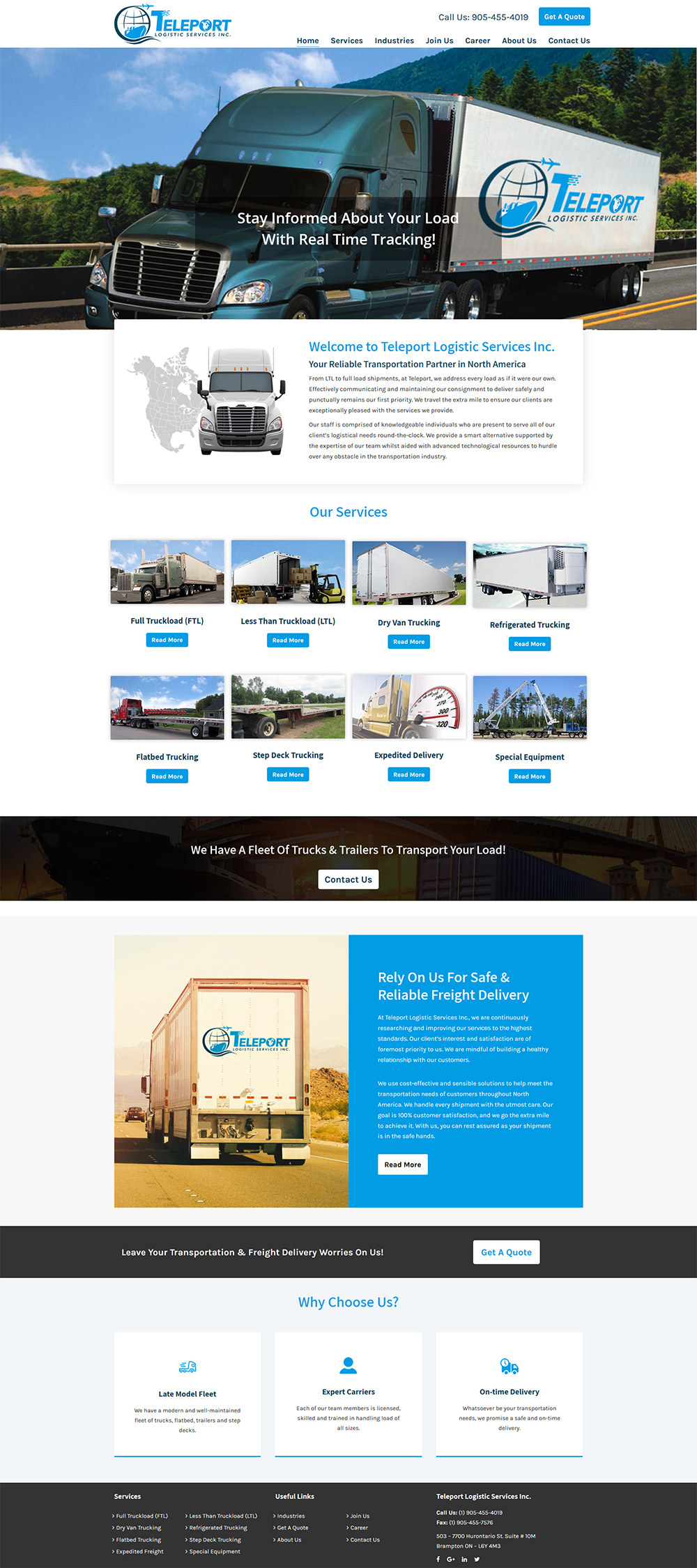**Landing Page of Teleport Logistics Services Inc.**

The landing page showcases Teleport Logistics Services Inc. and has been captured from a laptop, desktop, tablet, or smartphone. At the top, the page features a black silhouette of a globe with blue highlights at the bottom, alongside the company's name, "Teleport," prominently displayed.

The navigation menu at the top features dark blue clickable buttons with the options: Home (highlighted with a cyan underline indicating it is selected), Services, Industries, Join Us, Career, About Us, and Contact Us. Above this menu, there is contact information displaying "Call us: 905-455-4019" with a blue rectangular button reading "Get a Quote" in white text.

The central visual element is a semi-truck driving on a road under a blue sky with wisps of white clouds. The surrounding scene includes dark green trees and brown soil, with the semi-truck passing by a tan and black banister. The semi-truck itself is tan with a silver front, and the cargo bed is white, featuring the Teleport logo in silver. Yellow road lines accentuate the road scenery.

Adjacent to the truck image, a white rectangle illustrates the front view of a white semi-truck with a grey map of the United States behind it. On the right side, in blue text, it says "Welcome to Teleport Logistics Services Inc." Underneath, in dark blue, it reads, "Your reliable transportation partner in North America." Following this, in black text, it states:
"From LCL to full load shipments, at Teleport, we address every load as if it were our own. Effectively communicating and maintaining our consignment to driver safety and punctuality remains our first priority. We travel the extra mile to ensure our clients are exponentially pleased with the services we provide. Our staff is comprised of knowledgeable individuals who are present to serve all of our clients' logistical needs round-the-clock. We provide a smart alternative supported by the expertise of our team whilst aiding with the advanced technological resources to hurdle over any obstacle in the transportation industry."

The "Our Services" section, displayed in blue text, lists various offerings with corresponding images:
- A teal truck with a silver front and white back labeled "Full Truck Load (FTL)" and a blue "Read More" button.
- A truck being loaded, labeled "Less Than Truck Load (LTL)" with a "Read More" button.
- A truck positioned on a road, captioned "Dry Van Trucking" with a "Read More" button.
- An unhitched semi at the end of a road, labeled "Refrigerated Trucking" with a "Read More" button.
- A red and silver flatbed truck termed "Flatbed Trucking" with a "Read More" button.
- Another flatbed truck, this time for "Step Deck Trucking," with a "Read More" button.
- An AI rendition of a yellow and white semi-truck featuring a black and red speedometer reading "Expedited Delivery" with a "Read More" button.
- A crane positioned near a semi-truck, labeled "Special Equipment" with a "Read More" button.

This clean and structured layout visually and textually communicates Teleport Logistics' commitment to their clients and the variety of transportation services they offer.